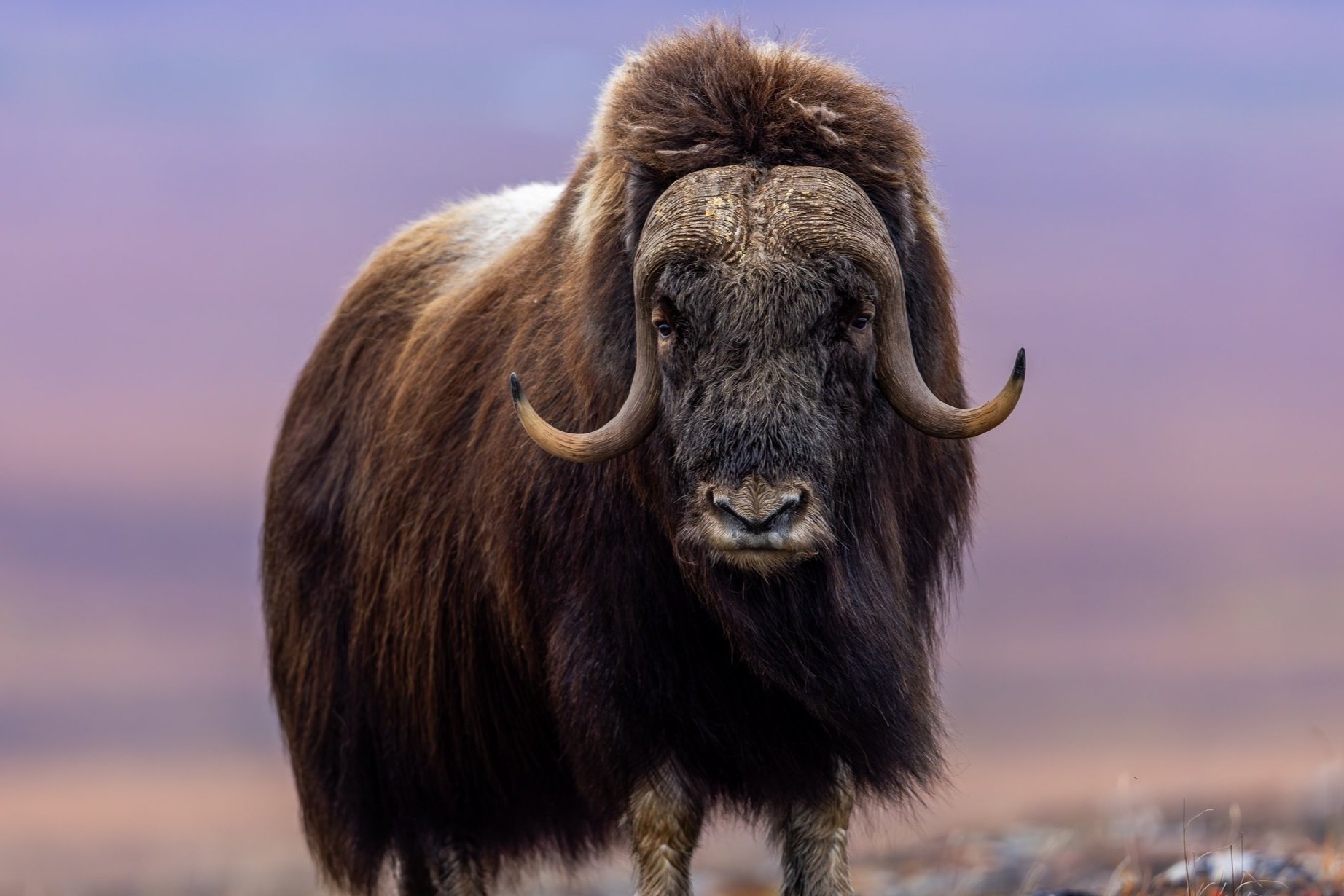The image depicts a realistic, horizontal artwork of a large water buffalo standing against a softly pastel pink and purple sky, which evokes the delicate light of dawn or dusk. The background is characterized by blurred, light-colored, fuzzy stripes, suggesting a dreamy sunrise or sunset. Positioned on the bottom right is a very muted and blurry area hinting at a rocky plain. The water buffalo stands with its rear facing the left side of the image and its head turned to gaze directly at the viewer, creating a striking centerpiece. Its long, shaggy coat is a mix of tan, rust, and dark brown hues, adding texture and depth to its massive frame. The buffalo's large head, about two feet by two feet, features two distinct, tan horns emerging from a central part, curving slightly upward along the sides of its face. The face itself is a darker gray interspersed with brown, while the snout combines shades of white, tan, and black. The soft depth of field blurs the animal’s back, emphasizing its imposing, grounded presence in the rocky landscape.